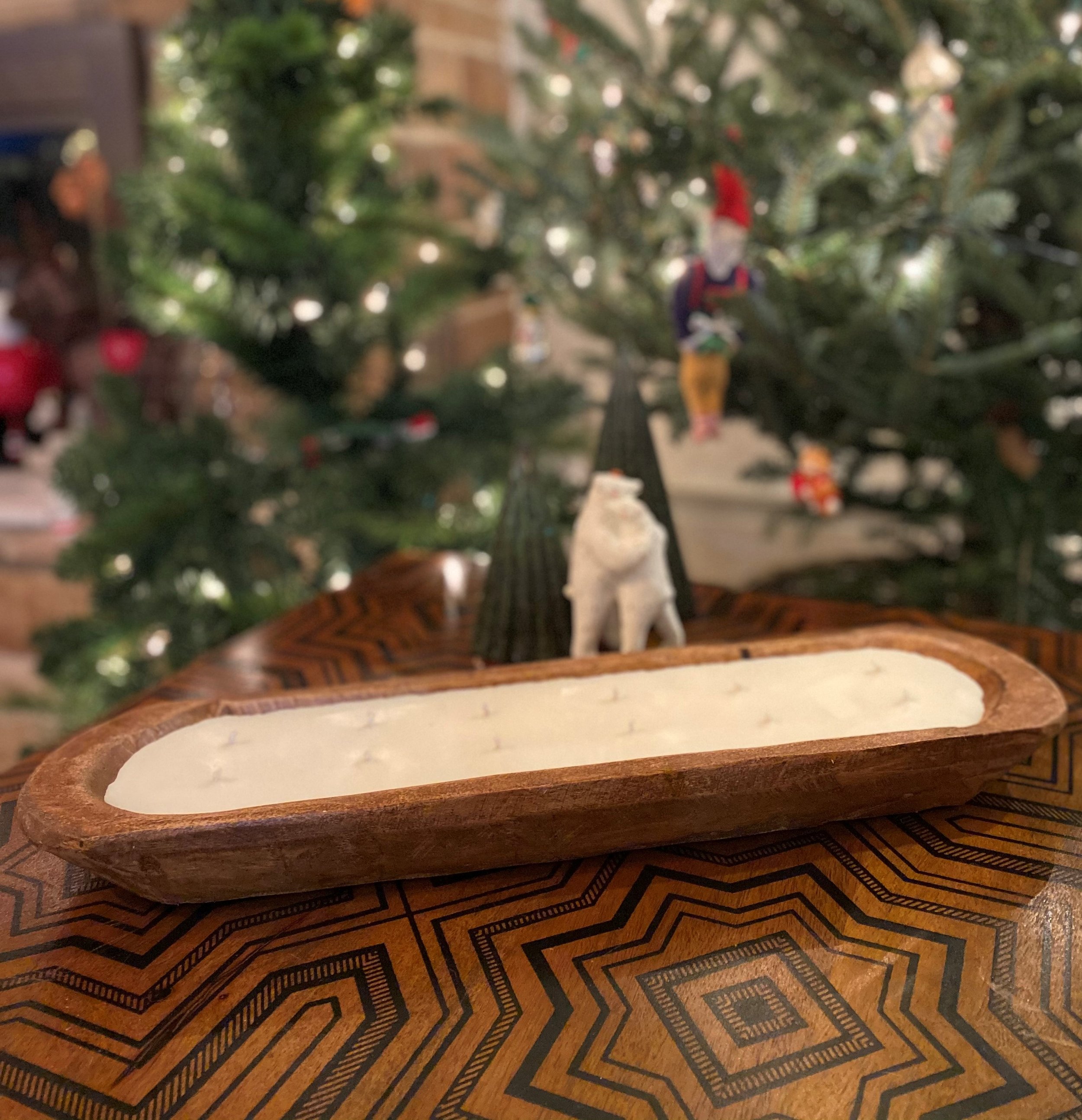This image showcases a close-up of a homemade candle set in a large rectangular bread bowl made of thick brown wood, showcasing its distinct wood grain texture throughout. The white handmade candle, unlit and featuring 12 pristine cotton wicks, sits atop a wooden table adorned with a detailed star pattern in varying sizes and borders. In the softly blurred background, festive elements such as a small white figurine and a lit Christmas tree can be discerned, adding a holiday ambiance to the scene.